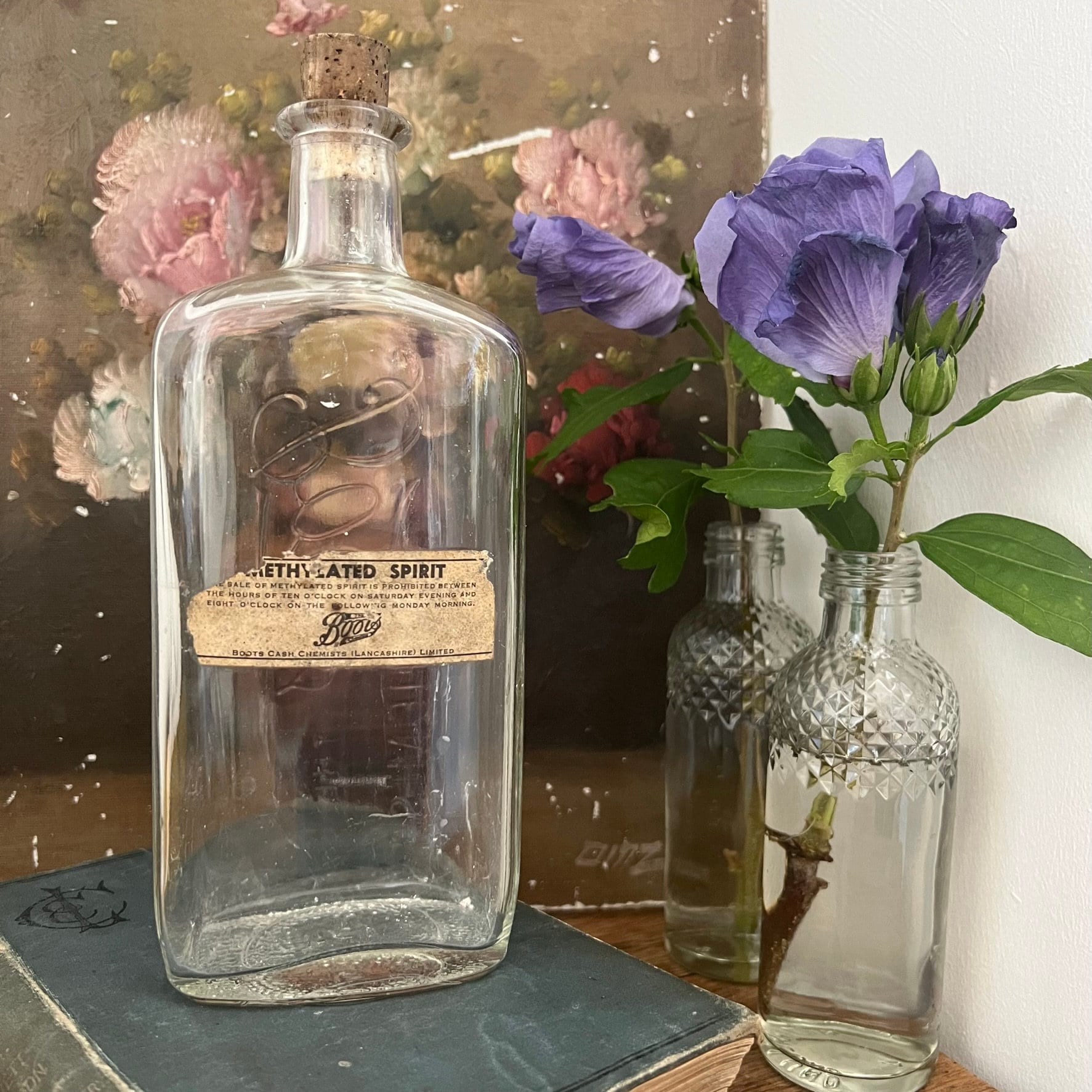The photograph showcases the top of a wooden table adorned with a collection of vintage and decorative items. Central to the image is an old, antique book with a blue cover, featuring a monogram in the top left corner that reads "L and C." Resting atop the book is an old, clear liquor bottle with a square base and a cork stopper. The bottle's partially torn label in black print reveals the words "methylated spirits" and a brand name that appears to be "Boots." Alongside the book and bottle, there are two decorative, clear jars, each with a twist spout and a diamond pattern running from midway up to the top. These jars, filled with water, serve as vases for beautiful purple flowers, possibly irises or lilacs. Completing the scene, leaning against a white wall at the back of the table, is a painting depicting flowers in a vase, adding a final touch of elegance and charm to the still-life arrangement.